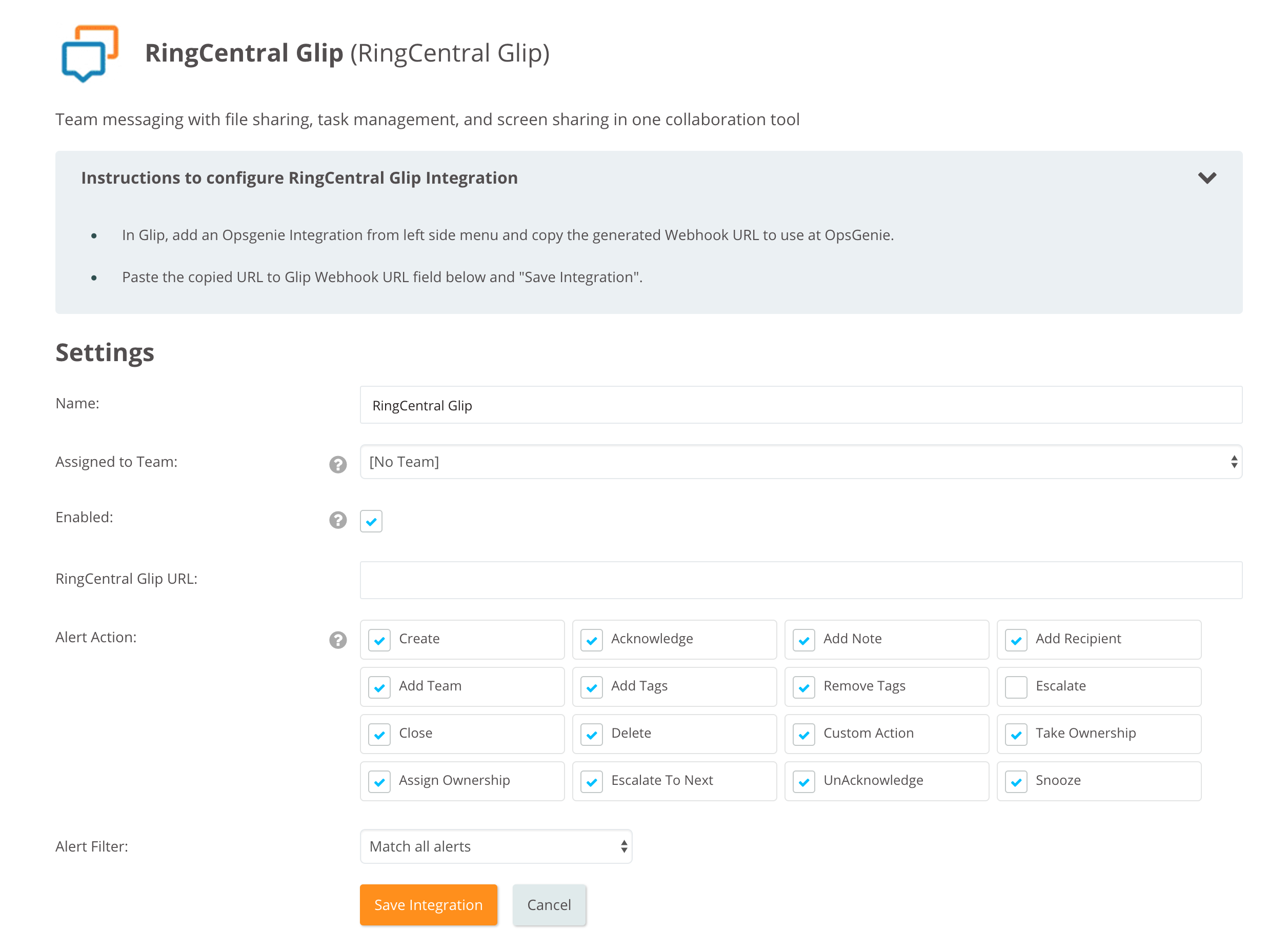**Detailed Descriptive Caption:**

A screenshot displaying the integration settings for RingCentral Glip within an OpsGenie interface. At the top, the interface title reads "RingCentral Glip" with an explanatory subtitle mentioning "Team messaging with file sharing, task management, and screen sharing in one collaboration tool." The next section provides step-by-step instructions on configuring the RingCentral Glip integration. Users are directed to add an OpsGenie integration from the left-side menu in Glip, copy the generated web hook URL, and paste it into the designated Glip URL field in OpsGenie before saving the integration.

Below the instructions, there's a heading labeled "Settings," which includes multiple configuration options: 

- **Name:** A field with a dropdown menu to assign a name.
- **Assign to Team:** Another dropdown to designate a specific team.
- The "Enabled" checkbox is marked to activate the integration.
- **RingCentral Glip URL:** A field to input the Glip URL.

The interface also includes a variety of alert actions, each with corresponding checkboxes. All actions listed—such as Create, Add Team, Close, Assign Ownership, Acknowledge, Add Tab, Delete, Escalate to Next, Add Note, Remove Tags, Custom Action, Unacknowledge, Add Recipient, Take Ownership, and Snooze—are enabled except for "Escalate."

At the bottom of the screen, users have the option to either "Save Integration" or "Cancel" the configuration.